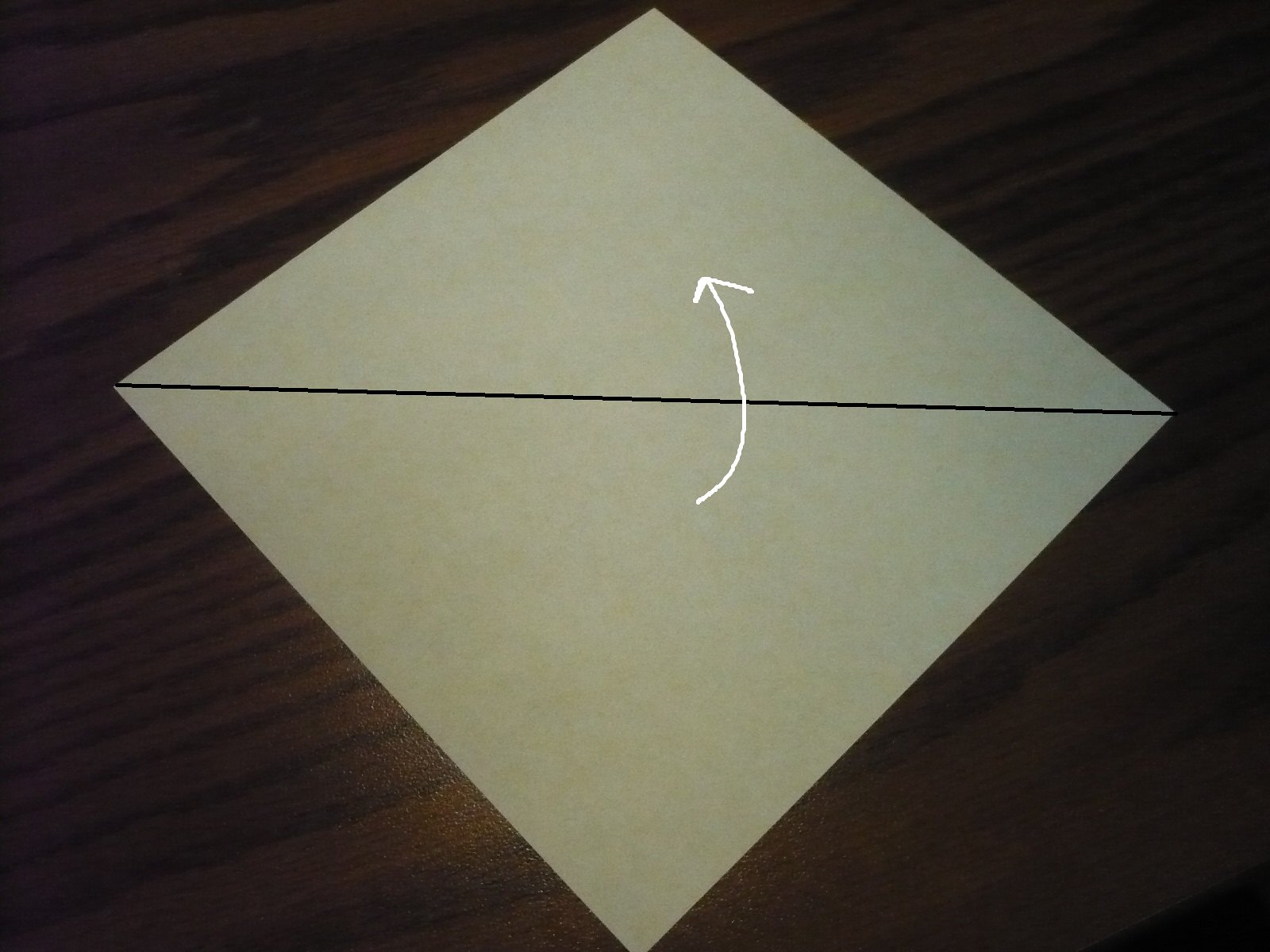A light gray square, slightly rotated to the left, dominates the image. A prominent black line crosses the square diagonally from one corner to the other, dividing it into two distinct triangles. Emerging from the center of the bottom edge is a hand-drawn, freehand arrow. This arrow curves upwards towards the right and then back towards the left, ending in a pointed tip that targets the center of the upper triangle. The square is placed on a dark brown wooden surface, which features diagonal lines running from the bottom left to the top right. The corners of the top triangles nearly touch the edges of the photo, while those on the side remain approximately an inch away.